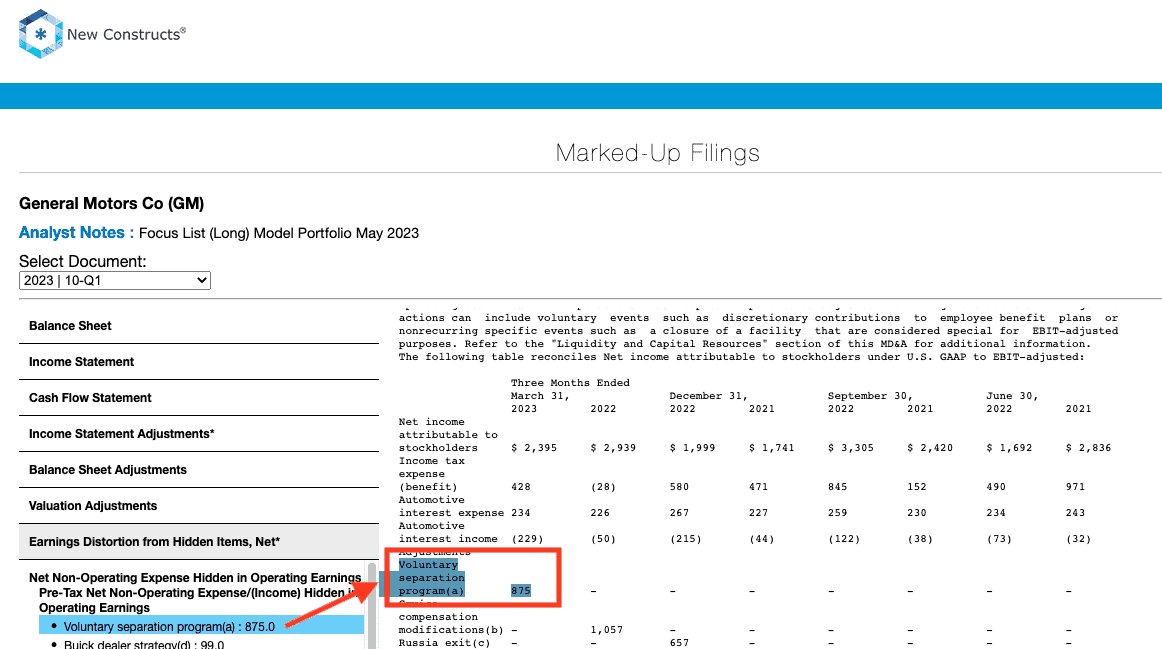The image, sourced from the website New Constructs, showcases a comprehensive financial document resembling a balance sheet or ledger. On the left side, a vertical menu lists various financial categories, including options to view the balance sheet, income statement, cash flow statement, and adjustments for income and balance sheets, among others. The right side features a detailed section filled with numerous figures and dates spanning from 2021 to 2023. The bottom right corner particularly highlights a budget-related entry titled “Voluntary Separation Program,” marked conspicuously in blue with the number 875 next to it. The document is presented in a clean format with black font against a white backdrop, ensuring readability and clarity.